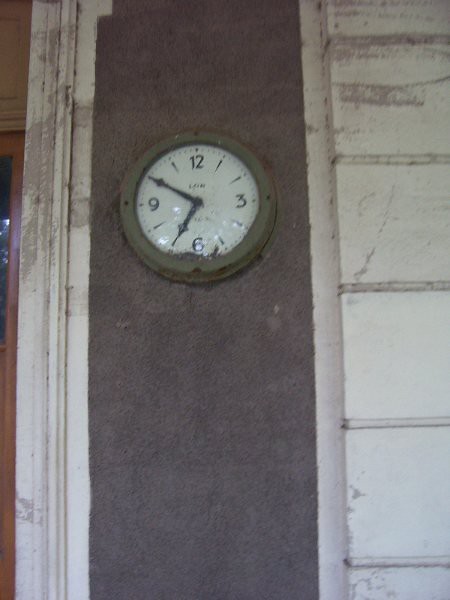This photograph captures a detailed scene of an outdoor clock mounted on a wall, which appears to be either on the exterior of a building or possibly in a garage setting. The clock itself is circular with a grayish-green, rust-spotted metal rim. Its face is white, featuring Arabic numerals at the 12, 3, 6, and 9 o'clock positions, and simple lines representing the remaining hours. Minute marks are indicated by dots. The clock hands are black, with the hour hand pointing to the 7 and the minute hand to the 10, displaying the time as 6:50. The clock is mounted on a section of taupe-colored trim. To its right, white horizontal siding, scuffed and dirty in parts, suggests an exterior wall, while to its left, the edge of a wooden doorway is just visible. Together, these elements create a visually engaging and detailed scene.